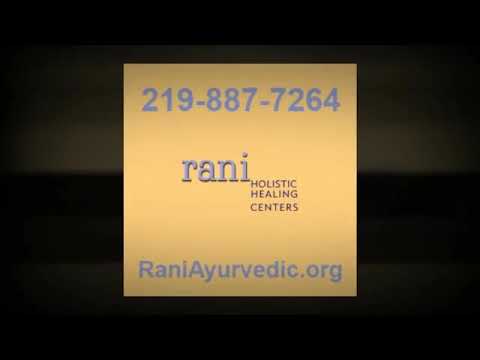The image features a prominent black border with a shaded effect, creating a subtle contrast between a darker black and a lighter black background. Within the center of the image is a gold square, reminiscent of a post-it note. At the top of this gold square is a phone number in blue letters: 219-887-7264. Underneath this, in the middle of the gold square, is the name "RANI" in large blue letters, followed by the phrase "Holistic Healing Centers," in smaller black letters directly beneath. At the bottom of the gold square is a web address, www.raniauyverdic.org, also in blue letters. The clean, structured arrangement of these elements highlights the advertisement for RANI Holistic Healing Centers, with the contrasting black border serving to draw focus to the gold square and its essential information.